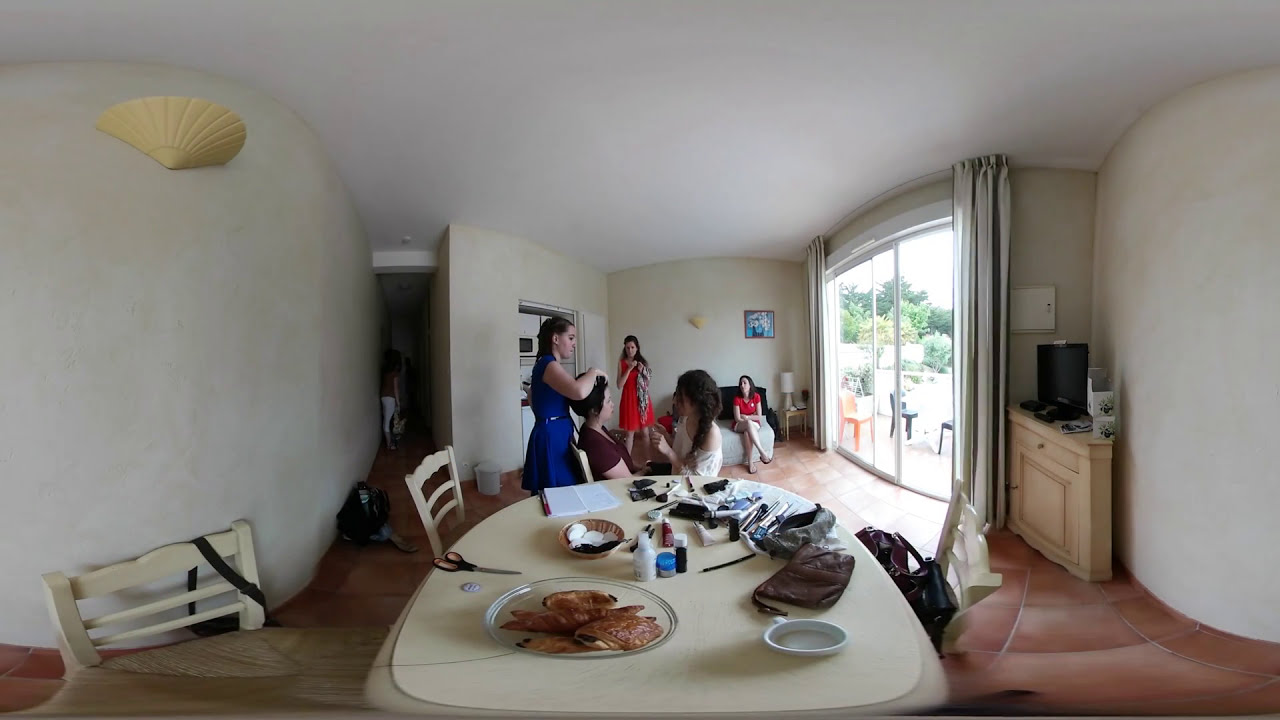This colorful, panoramic indoor photograph, likely taken with a fisheye lens to create a slightly distorted and curved effect, captures a detailed scene of a group of young women in what looks to be a living area of a house or apartment during daytime. The room is lit by natural daylight filtering through an open pair of large white sliding glass doors on the right, leading to a balcony or porch area. The floor is covered in brown tiles, and the walls and ceiling are painted white.

In the foreground stands a white table cluttered with various personal items—a cup, a plate of food that appears to include chicken or toast, a pair of scissors, two purses with contents spilled out, a bowl of pastries, and a notepad. 

To the left of the table, two women are interacting; one, dressed in a blue dress with long hair, stands over another woman seated in front of her wearing a maroon shirt. The woman in blue seems to be working on the hair of the seated woman. To their right, another woman is dressed in white with dark brown hair, observing the scene. 

Further in the background, near a bed with a bedside table and lamp, are two more women; one stands wearing a red dress, while the other, dressed in a red top and brown pants, sits on the edge of the bed. Additionally, there's a tabletop partially visible with miscellaneous items on it to the right of the sliding glass door.

On the left side of the image, a darker hallway stretches back, where two indistinct figures can be seen, adding depth to the bustling atmosphere of the room.